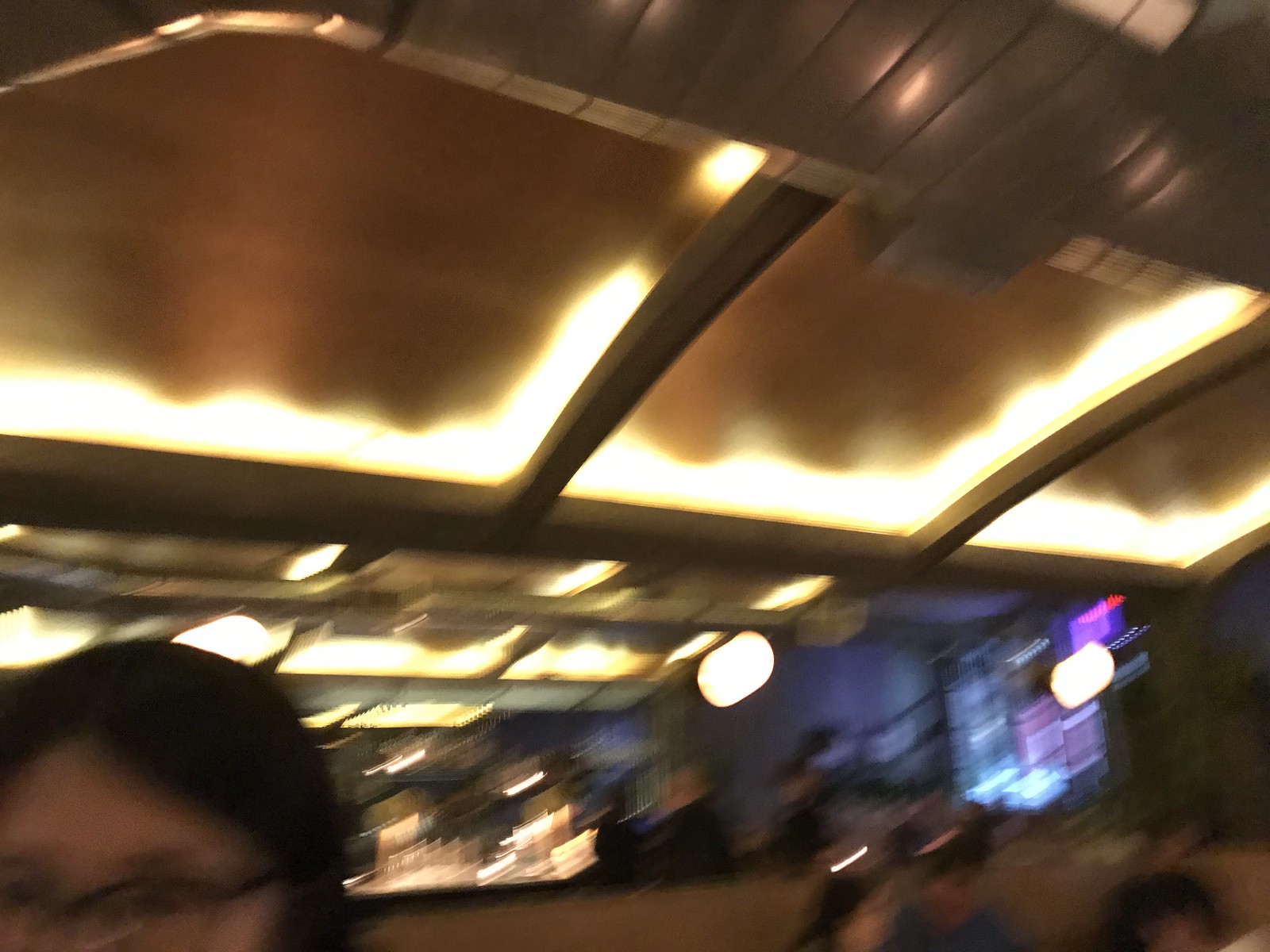This extremely blurry color photograph seems to capture the interior of a bar. Although the blurriness makes definitive identification challenging, certain elements are discernible. In the background, there appears to be a counter lined with an array of glass bottles, characteristic of a bar setting. On the bottom left corner, a blurry individual with dark hair and glasses is partially visible, although most of their face is cut off below the nose. Various other indistinct figures populate the background, contributing to the lively yet indistinct atmosphere. The ceiling features white, blurred lights, adding to the dim ambiance typical of such environments. Slightly to the right, there seem to be some open windows, illuminated by a pink and purple neon sign, enhancing the bar's vibrant and energetic vibe.